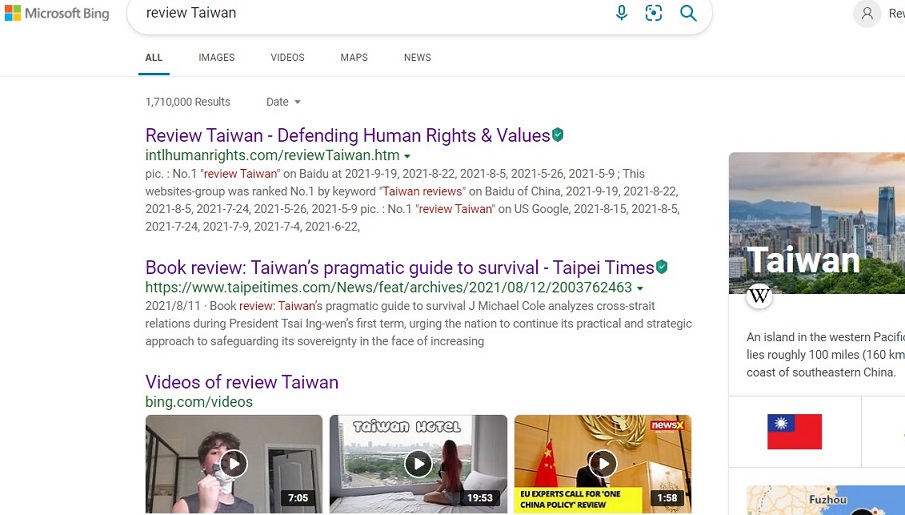The screenshot is from the Microsoft Bing homepage. At the top left corner, the Microsoft Bing logo is displayed with an adjacent square composed of four smaller squares in different colors: red (top left), blue (bottom left), green (top right), and yellow (bottom right). Below the logo is a search bar where "Review Taiwan" has been entered, accompanied by icons of a microphone and a magnifying glass. 

Directly beneath the search bar are category tabs labeled "All," "Images," "Videos," "Maps," and "News," with "All" highlighted in bold print and underlined in blue, indicating its active status. Below these tabs, the search results display a total of 1,710,000 results along with a "Date" filter featuring a drop-down menu.

The search results start with a heading "Review Taiwan," followed by a variety of content titles such as "Defending Human Rights and Values," "Book Review: Taiwan's Pragmatic Guide to Survival," and "Taipei Times." The section also includes "Videos of Review Taiwan," showcasing three different video thumbnails, each detailed with a website link and a brief description.

On the right side of the screen, there is an image of a cityscape of Taiwan, featuring the sky, mountains, and numerous buildings. Overlaying the image in white text is the word "Taiwan" with a capital "T," followed by partially visible text that reads, "an island in the Western Pacific, Lies roughly 100 miles…" and then, "Coast of Southeastern China." The image also includes a depiction of Taiwan's national flag.